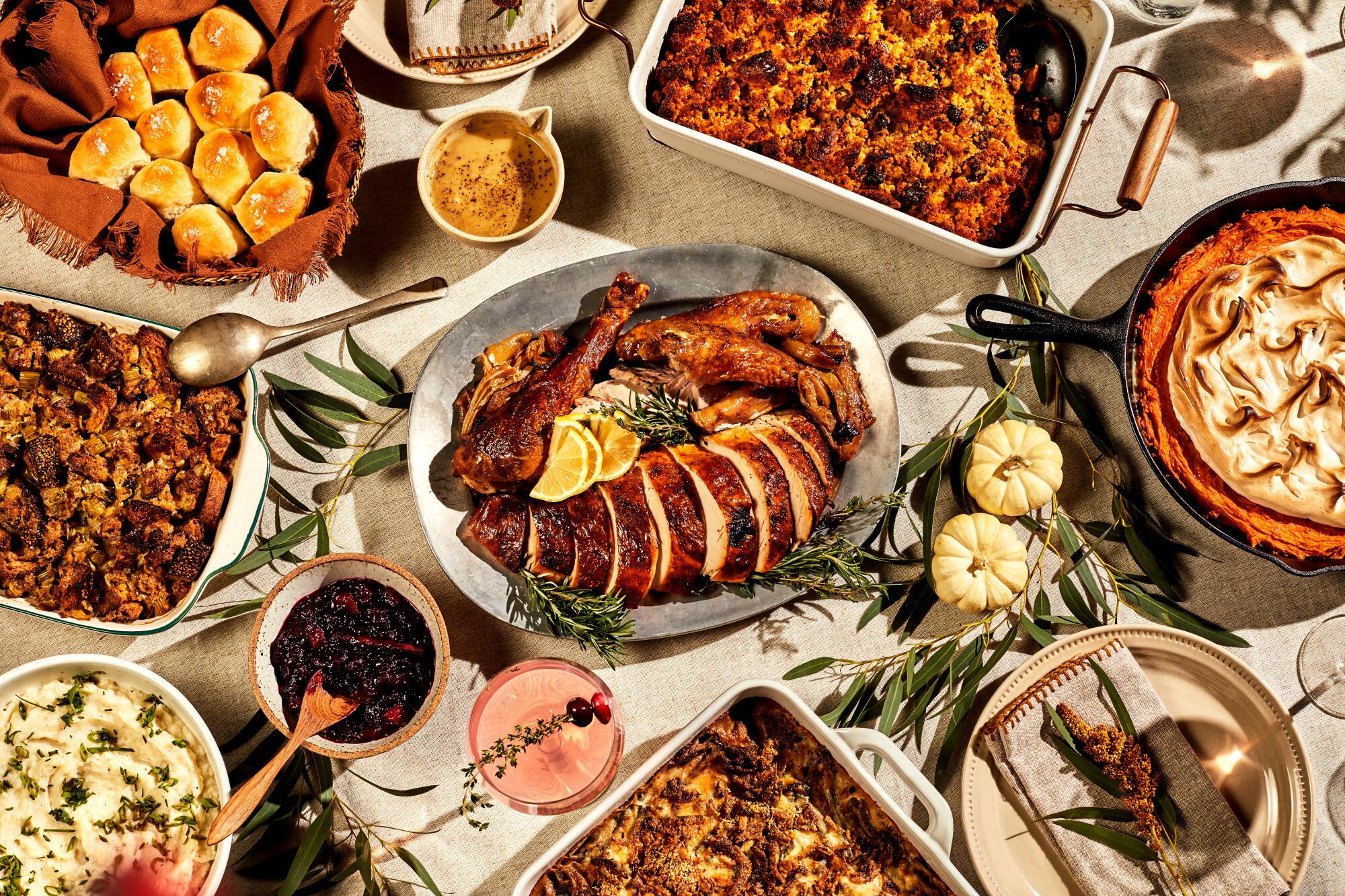This detailed overhead image showcases an abundant spread of approximately ten dishes, artfully arranged atop a cream-colored tablecloth embellished with green leafy garnishes and small white pumpkins. Starting from the upper left and moving clockwise, the table features a basket lined with a brown cloth, holding about 10 to 12 golden bread rolls. Adjacent to it is a small white circular container of brown gravy. A white casserole dish, likely containing sweet potato casserole or pie with a meringue topping, sits nearby.

In the central portion of the image, an oval silver platter prominently displays accordioned slices of meat, possibly chicken or turkey, garnished with lemon wedges and green sprigs. Surrounding this centerpiece, the arrangement continues with various dishes: a white circular bowl of mashed potatoes is situated in the bottom left corner, next to a circular container of red cranberry sauce. Further along, another white casserole dish is visible, along with other dishes including what looks to be bread stuffing, and skewers of food.

Additionally, a drink garnished with a slice of fruit, likely an orange, can be seen among the dishes. The diverse array of bakeware, ceramic pans, cast iron skillets, and silver platters collectively present a bountiful and visually appealing feast.